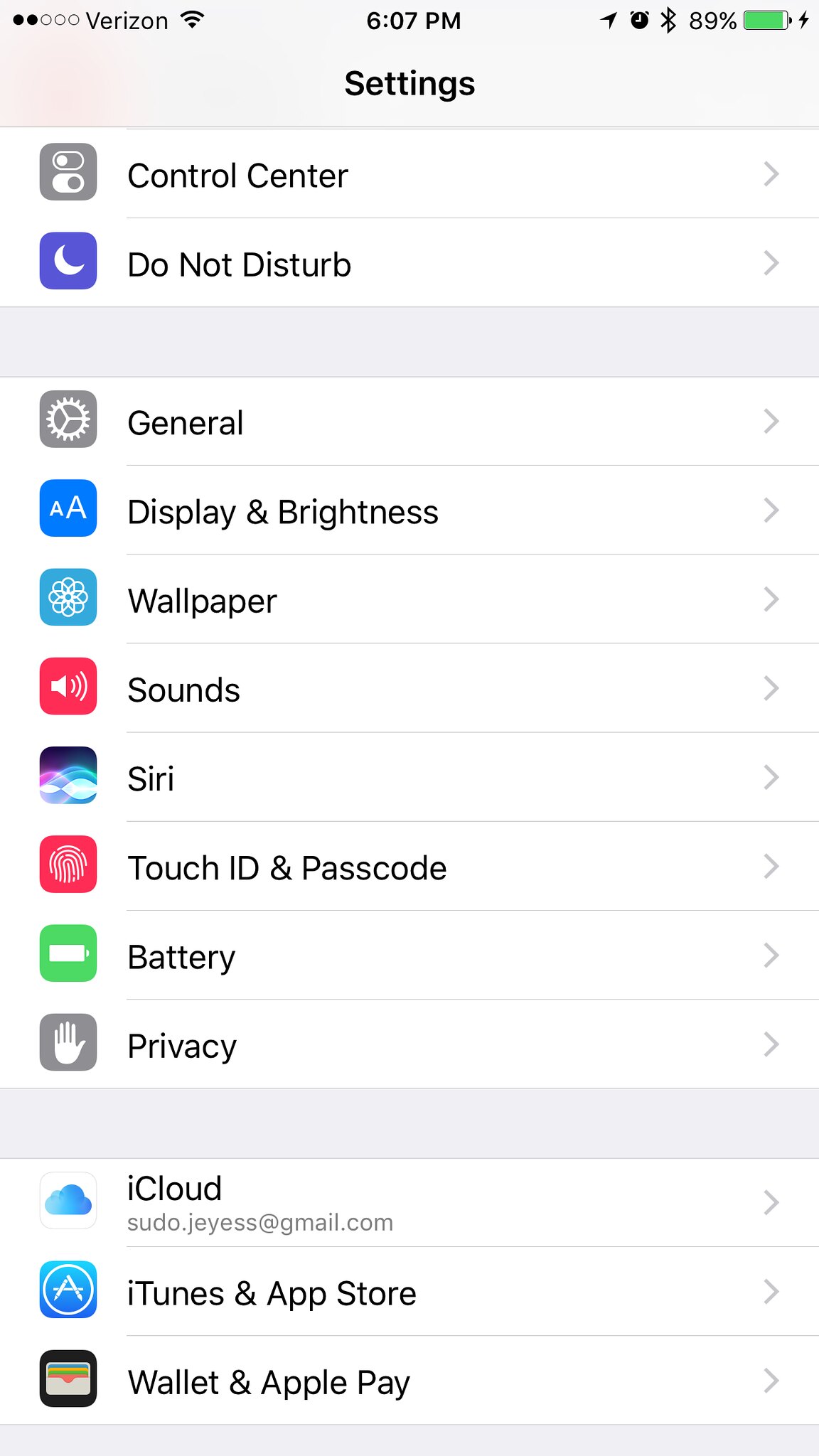Screenshot of an iPhone Settings Page:

At the top left corner of the screen, the status bar displays "Verizon" with a Wi-Fi signal and a partial cellular signal (two out of five bars). In the middle of the top bar, it shows the time as 6:07 p.m. On the right side, there are icons for location services (a small clock), Bluetooth, and a battery indicator showing 89% power, currently charging (indicated by a green battery icon with a lightning bolt next to it).

Just under the status bar, the title "Settings" is centered at the top of the screen. Below the title, there is a vertical list of menu items, each contained within a white rectangle. The menu items and their accompanying icons are as follows:

1. **Control Center**
2. **Do Not Disturb** - represented by a blue square with a white crescent moon.
3. **General** - indicated with a gray square featuring a white gear wheel.
4. **Display & Brightness** - shown with a blue square and two white "A"s of different sizes.
5. **Wallpaper** - symbolized by a blue square with a swirly graphic design.
6. **Sounds** - marked by a red square with a white speaker icon.
7. **Siri & Search** - displayed with a black square featuring the colorful Siri animation.
8. **Touch ID & Passcode** - indicated by a red square with a white fingerprint icon.
9. **Battery** - represented by a green square with a white battery icon.
10. **Privacy** - symbolized by a gray square with a white hand icon.
11. **iCloud** - indicated by a white square with a blue cloud icon, displaying the email address "sudo.jssoju-yess@gmail.com" beneath it.
12. **iTunes & App Store** - shown with a blue square that contains the App Store icon.
13. **Wallet & Apple Pay** - represented by a black square with a small card case icon.

This detailed summary encapsulates the visual elements of the screenshot, highlighting the hierarchical structure and unique icons associated with each setting option.